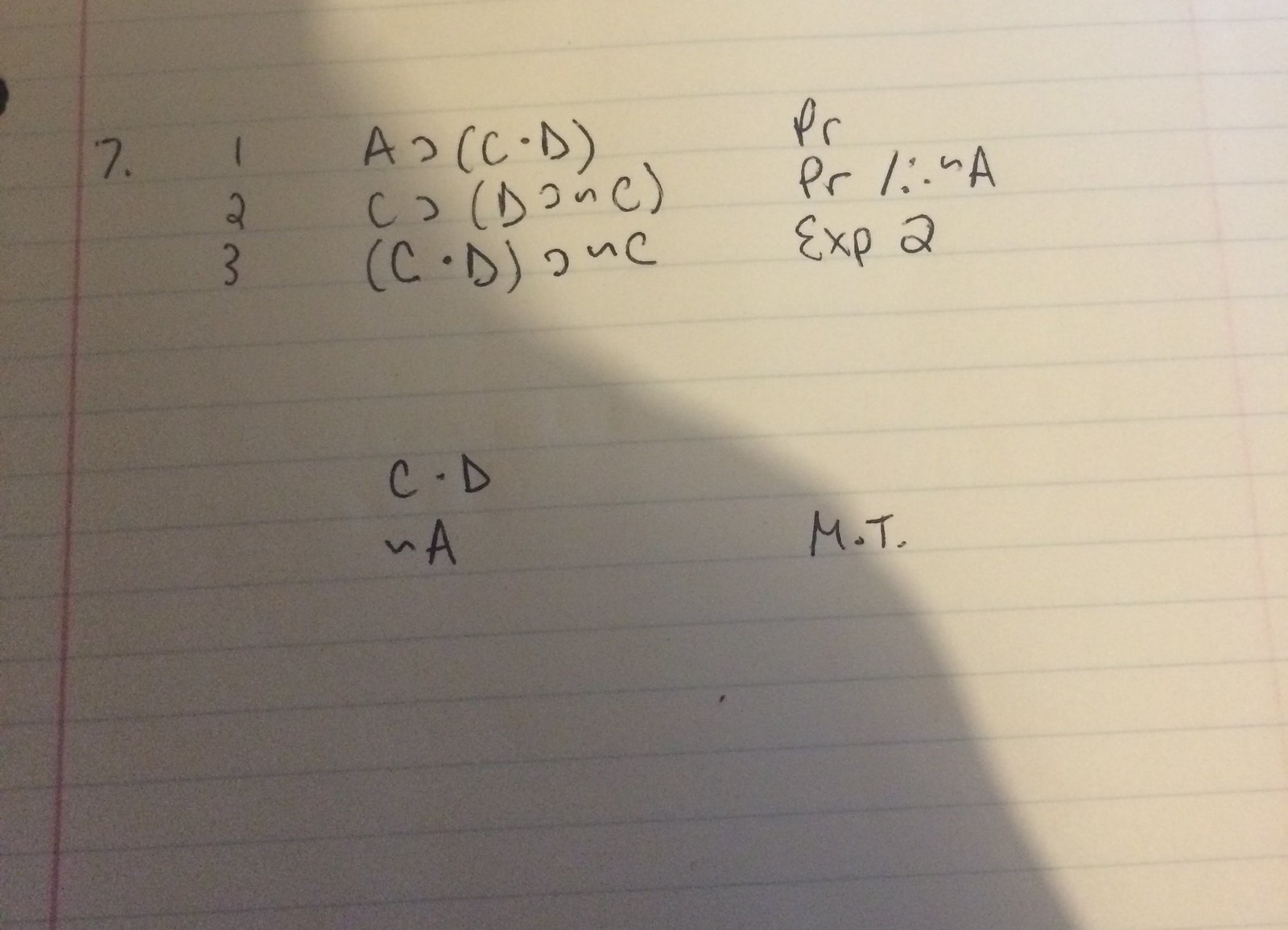In the image, there is a photograph of an old, slightly tattered piece of college-ruled lined paper containing a written math assignment. The assignment appears to be part of a numbered series, as the top left corner has a bold "7" indicating it is problem number 7. The detailed handwritten equations and notations suggest a mathematical exercise that is somewhat advanced.

On the first line of the assignment, it reads "1: A and (C - D) PR," although the exact mathematical context of "PR" is unclear. A subsequent line labeled "2" shows another equation: possibly "(D and C)" though the symbols are difficult to interpret precisely without further context.

Moving down to the third line, it states: "C - D EXP2," which might indicate an operation involving exponents, specifically the square of (C - D). At the bottom of the page, there is a final line reiterating "C - D," followed by the notation "M.T." which could stand for a specific method or mathematical technique, though its precise meaning remains ambiguous.

The entire page reflects typical elements found in handwritten homework: meticulous step-by-step problem-solving, though the exact type of mathematics is not immediately recognizable. The hand-drawn nature of the work adds a personal touch, indicative of a diligent student working through complex math problems.